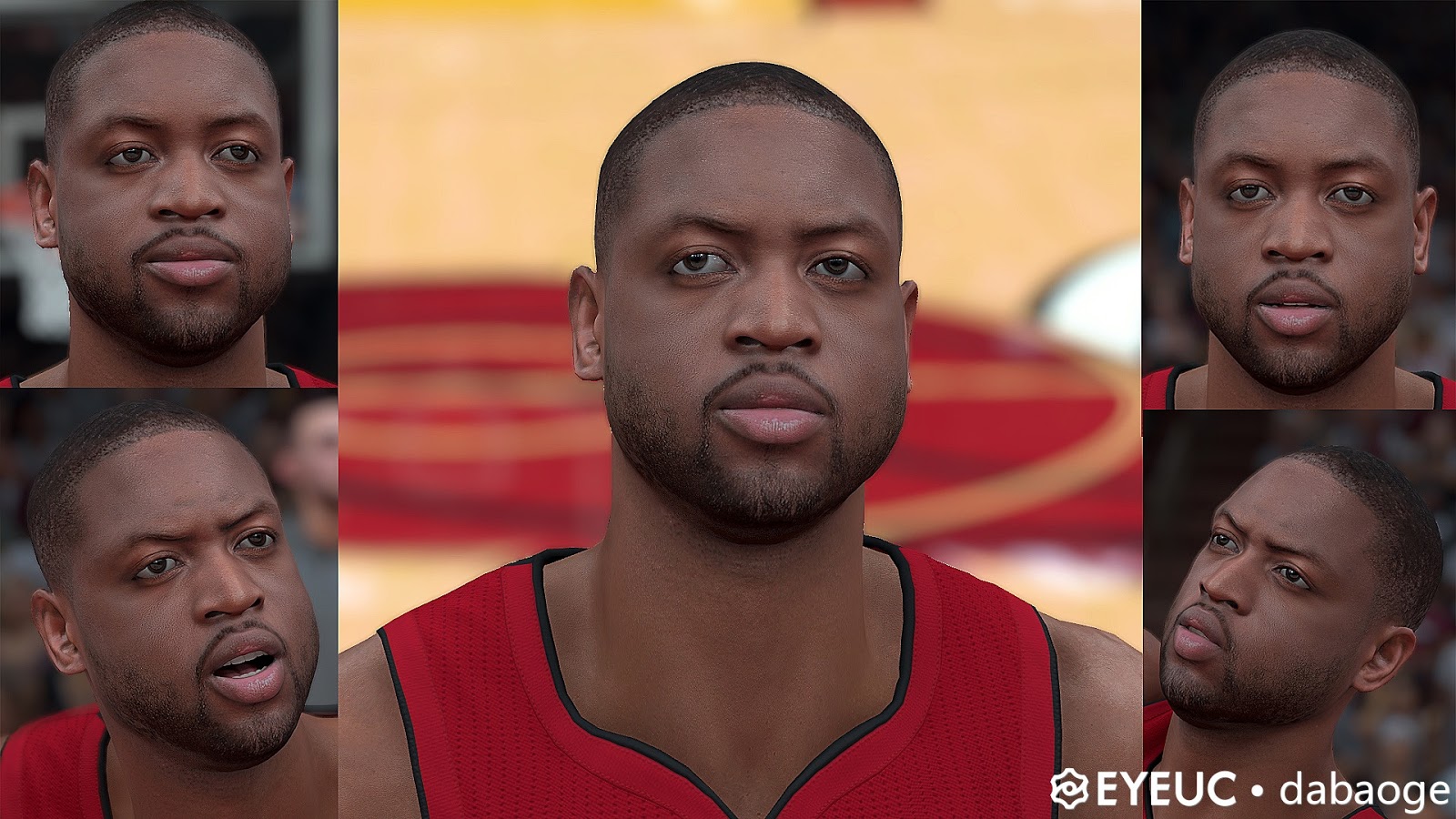The image showcases a collage of five screenshots from a video game, all featuring the same character: a Black man with very short hair, a thin beard, and mustache, complemented by sunken eyes and a prominent nose. The layout consists of four smaller pictures surrounding a larger central one. The background of these images varies from a dark hue to a crowd scene.

1. **Upper Left Image**: The man is looking slightly to the right. A red shirt is partially visible at the bottom right corner.
2. **Upper Right Image**: The man faces straight ahead, with a red shirt visible on both shoulders.
3. **Lower Left Image**: The man appears extremely confused, looking to the right, and more of the red shirt is visible.
4. **Lower Right Image**: The man looks to the left with a serious-yet-confused expression.

The central image features a tan-and-red background, likely depicting a basketball court, with a clearer view of the man’s jersey outlined in black. A caption in the bottom right reads, "E-Y-E-U-C. D-A-B-A-O-G-E."